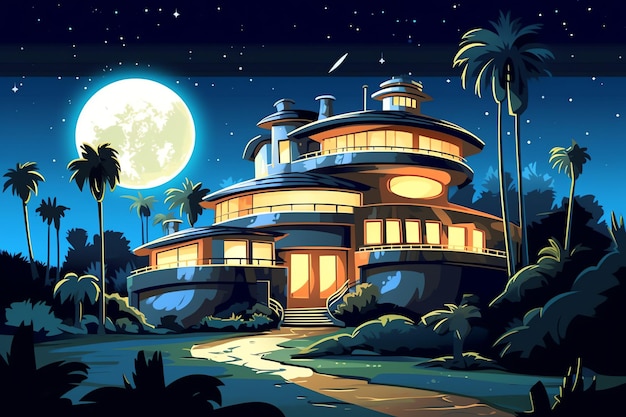The illustrated nighttime image features a very modern, multi-story home depicted in a cartoon style. The backdrop transitions from a lighter blue at the horizon to a dark, almost black sky at the top, dotted with numerous white stars. A full moon dominates the sky to the left of the house, casting a serene glow. A shooting star is visible near the top center, adding a whimsical touch.

The house itself is an architectural marvel with a cylindrical and circular build, spread across several levels. From the top, a small lookout tower descends to a room encircled by a deck and railing, then down to a level with expansive windows and railings. Below this, there are smaller windows and doors, leading down to a grand entrance with a front door flanked by a staircase. A side room with two doors further enhances the complexity of the structure. 

Palm trees and lush tropical vegetation surround the house, creating an exotic atmosphere reminiscent of locations like the Hollywood Hills in California. A rock or dirt pathway, framed by freshly mowed grass, leads invitingly up to the front steps of the home, suggesting a well-maintained and vibrant environment. The overall scene is lively and enchanting, illuminated against the tranquil night sky.